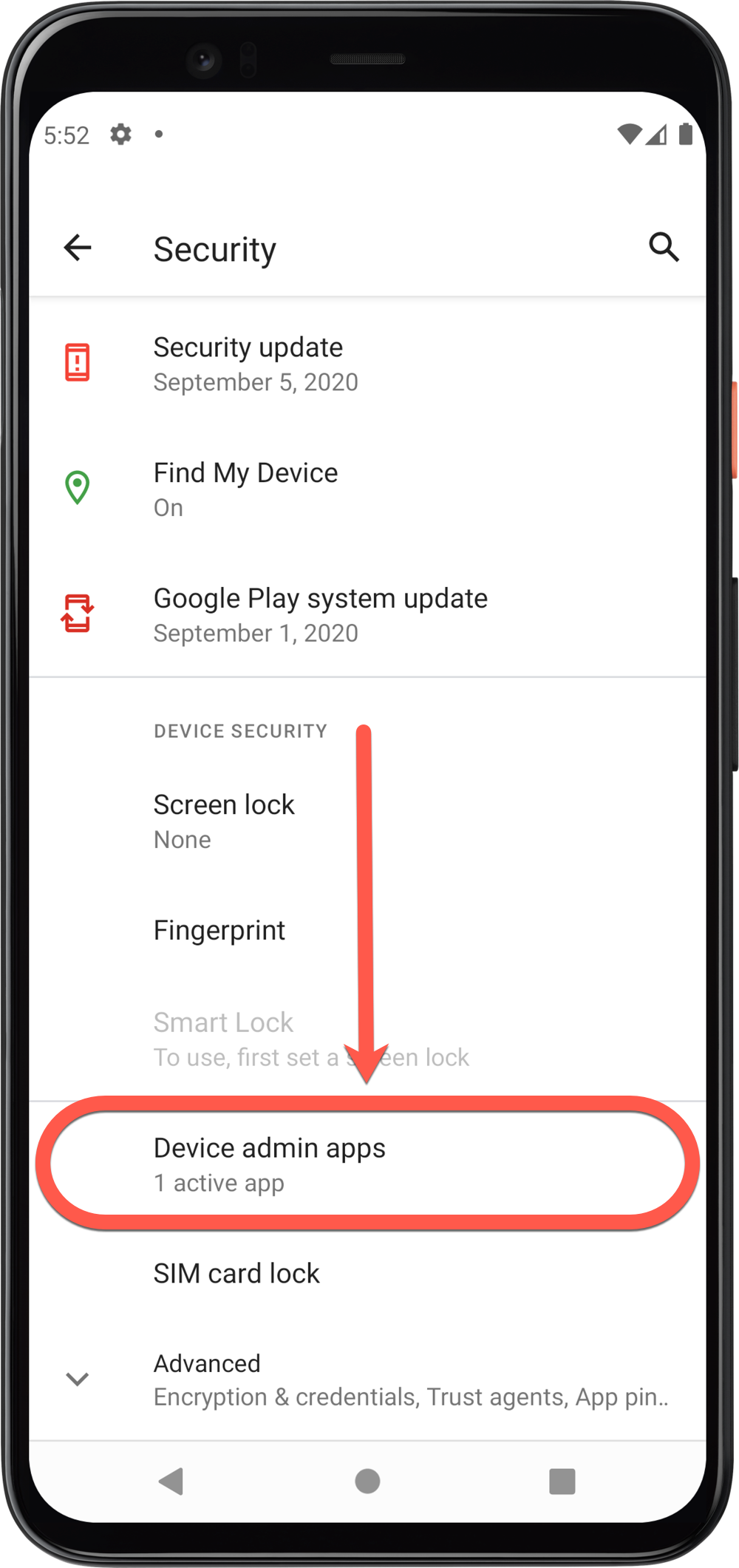The image is a detailed screenshot taken from a smartphone, where the phone itself is visible around the edges of the screenshot, creating a black border against the white screen interface. The phone's status bar at the top displays the time as 5:52, a full battery icon, and half signal strength.

The main content of the screenshot falls under the "Security" settings section. It begins with a notification indicating that a security update took place on September 5th, 2020. Below this, it states that the "Find My Device" feature is enabled, and that the Google Play system was last updated on September 1st, 2020.

Further down, under "Device security," it shows that no screen lock or fingerprint authentication has been set up. The "Smart Lock" function is mentioned but is displayed in very faint, hard-to-read text, suggesting it is not recommended or emphasized.

A prominent red ring encircles the "Device administrative apps" section, with a large red arrow pointing down to highlight its presence. This section indicates that there is one active app with administrative privileges.

Following this, there is an option for "SIM card lock," and an "Advanced" category containing settings for "Encryption and credentials," "Trust agents," and "App pinning." The screenshot concludes here, representing a comprehensive overview of the current device security settings.